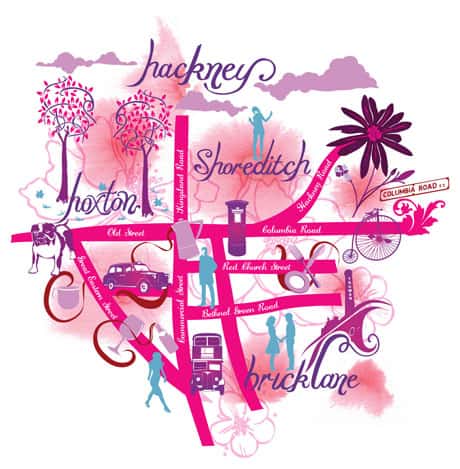This is a vibrant, computer-designed street map set on a white background, dominated by shades of pink. The map is marked with bright pink streets that carry names in flowing white script. The top-left corner features two purple trees with a horse stand nestled between them. Below this, a triangular section framed by three streets houses a purple car. Prominently, the turquoise label "Hackney" adorns the top, followed by "Shoreditch" and "Hoxton" further below. The lower section of the map features a dog, a purple cup, a purple glass, and a blue lady walking. At the bottom, a purple double-decker bus is positioned between two streets, with a blue couple facing each other to its right, above the inscription "Brick Lane." Other notable illustrations include an old-style black taxi, a London phone booth, and a vintage penny-farthing bicycle near Columbia Road on the right. Additionally, the map artistically includes a scattering of turquoise human silhouettes, enhancing its stylized representation of urban life.